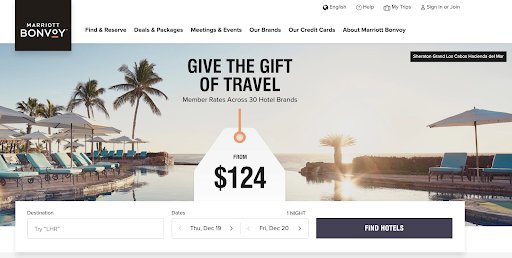The top of the image prominently features the "Marriott Bonvoy" logo, alongside navigation options such as "Find & Reserve," "Deals and Packages," "Meetings & Events," "Our Brands," "Our Credit Cards," and "About Marriott Bonvoy." Language selection is set to English, and user options include "Hello," "My Account," "Sign In," and "Join."

The image promotes Marriott Bonvoy's offering, highlighting travel rates across 30 hotel brands, starting from $124. A city destination and flexible date selections (Thursday, December 19th to Friday, December 29th) suggest a vacation planning theme, with a "Find Hotels" button inviting further exploration.

The scenic view features a beach setting with several chairs and umbrellas arranged along the shoreline. Palm trees with lush green leaves frame the background, along with the shimmering water reflecting the sun. The idyllic beach setup includes additional chairs and umbrellas closer to the water's edge, with more palm trees and some decorative stone structures enhancing the tropical paradise ambiance.